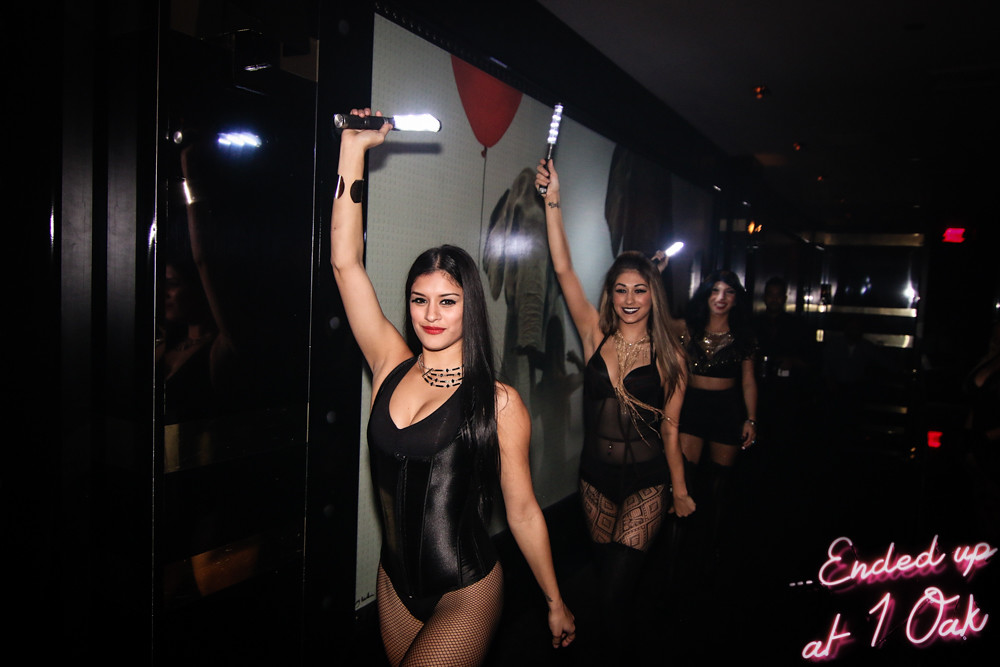In this wide and slightly desaturated photograph, three women dressed in black unitards and sheer tights are walking towards the camera, though slightly angled to the right. Each woman holds a small portable light aloft, casting a faint glow in the otherwise dimly lit room. The woman in the front, positioned slightly left of center, sports a black leotard, a four-string black choker, and lets her long dark hair fall in front of her. Following her, the second woman’s long blonde hair and the third woman’s similar attire and light-holding pose create a sense of uniformity. They walk against a dark wall adorned with a subtle mural of an elephant and a red balloon, though details remain obscured due to low lighting. Script text in the lower right corner, glowing white with a pink halo, reads "ended up at one oak." A faint, indistinct male face is visible in the distance behind the last woman.